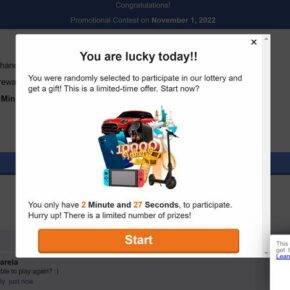The website features a prominently blue and white themed background design, segmented into two blue strips framing a central white section. At the top of the page, a bold headline reads "Congratulations" above an announcement for a promotional contest dated November 1, 2022. Centrally placed on the page is an open box graphic with the message, "You are lucky today," inviting the viewer with the text, "You were randomly selected to participate in our lottery and get a gift. This is a limited time offer, start now."

Beneath this message, a photo collage showcases an array of enticing prizes jumbled together in a cluster, including a car, the number "10,000," a black scooter, a Game Boy Switch, and various other indistinguishable objects obscured by overlapping items.

A countdown timer below the image urges participation within "two minutes and 27 seconds" and highlights the scarcity of available prizes. At the bottom of the white section, a long orange bar labeled "Start" beckons viewers to take immediate action.